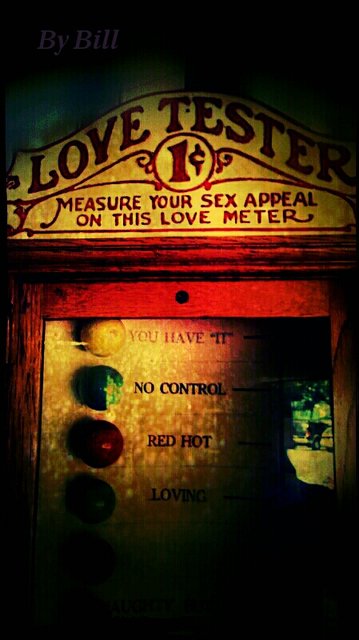This photograph features a vintage Love Tester machine, often seen at fairs and carnivals, set against a dark background. The top of the machine showcases a white, arched cap with curved red lettering that reads "Love Tester." Beneath this, a white circle outlined in red displays the cost "1¢." Below, the text in red on a white background instructs, "Measure your sex appeal on this Love Meter." The machine is encased in a reddish wooden frame, which holds a series of colorful buttons. The top yellow button is labeled "You Have 'It'", followed by a green button with the text "No Control," and a red button reading "Red Hot." As the image fades into darkness at the bottom, another button is partially visible, suspected to read "Love." To the left of each text label is a corresponding colored circle, possibly resembling gems.